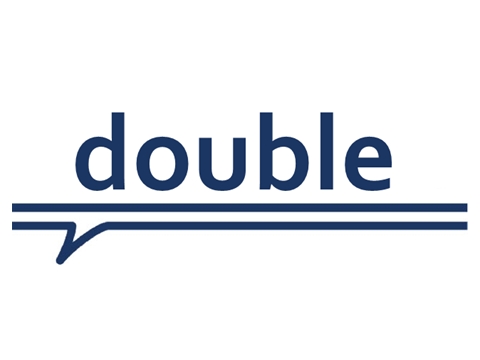The image features a clean and modern logo with the word "double" prominently centered in lowercase, sans-serif font in a dark navy blue. Beneath the word "double," there are two distinct horizontal lines. The first line is a simple, straight line extending horizontally beyond the word "double" in both directions. The second line, of the same length, has a subtle V-shaped indentation pointing downward in the middle, reminiscent of a division or square root symbol. The entire logo is set against a clear white background, ensuring high clarity and ease of visibility, making it suitable for various business or small company branding.